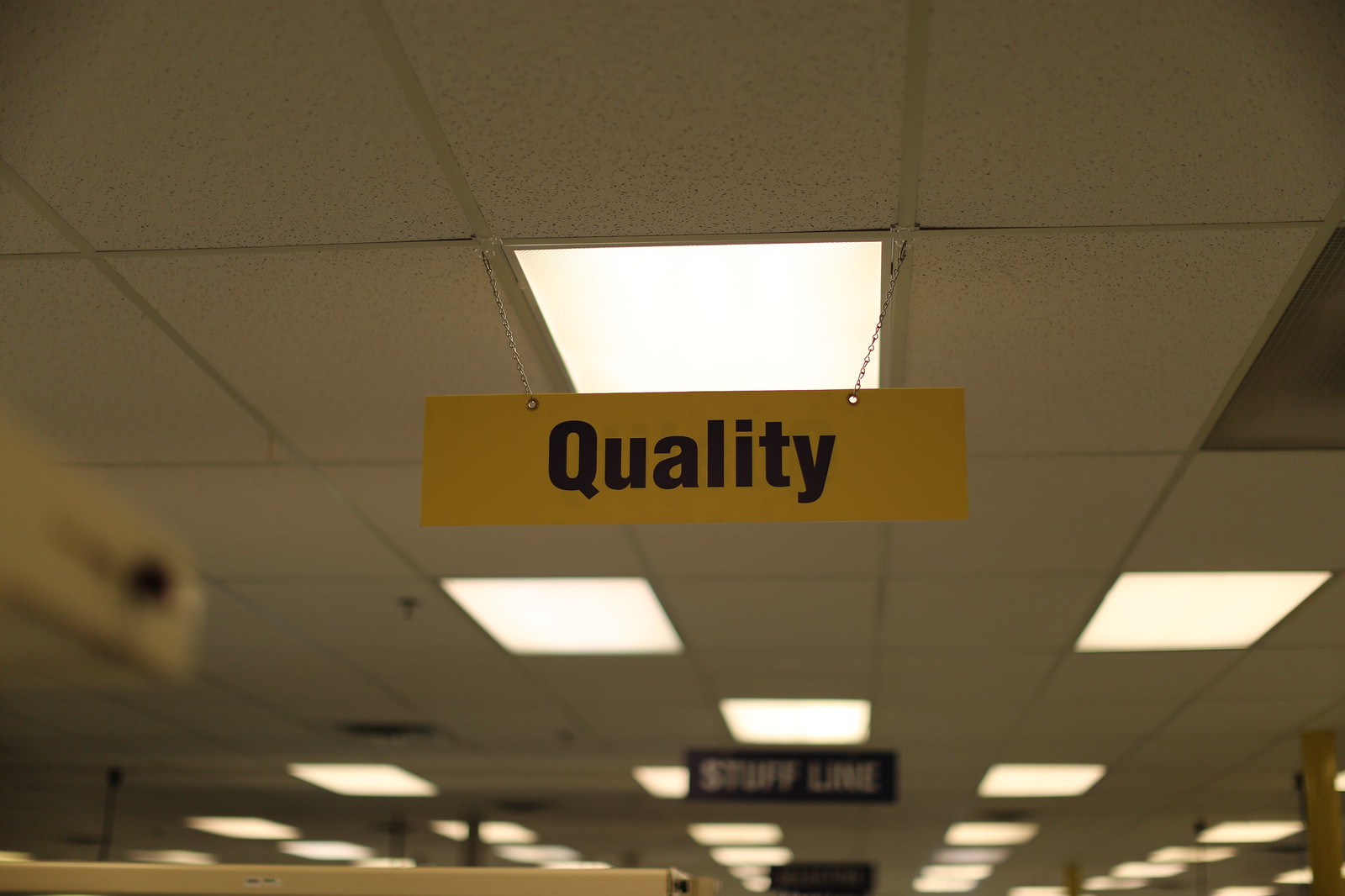The image captures a view looking up towards the ceiling of what appears to be a retail establishment or office space. The ceiling is composed of white rectangular planks arranged in a drop ceiling grid, interspersed with fluorescent light panels. Prominently hanging in the foreground from silver chains attached to the ceiling grid is a mustard yellow rectangular sign with black text reading "Quality." The background is slightly blurred, but another sign can be seen a few panels down, which appears to be black with white text, possibly reading "Staff Line." Some ceiling tiles are missing, contributing to the perception of a skylight effect. The overall scene suggests an organized, grid-like ceiling layout typical of an office or commercial environment.